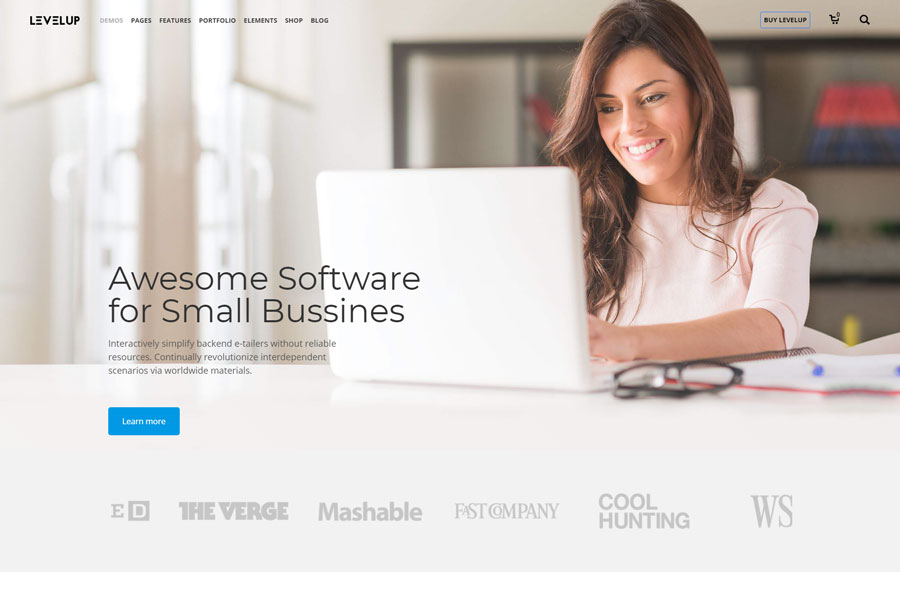The image is a detailed screenshot of a laptop screen displaying information about a software company named Level Up. Their black logo is positioned in the upper left corner of the image. In the center, a fair-skinned woman with long, wavy brown hair is seated in front of a white laptop, smiling warmly. She wears a pink blouse with elbow-length sleeves. The blouse has the text, "Awesome Software for Small Businesses," printed on it, followed by a smaller description: "Interactively simplify back-end e-tailers without reliable resources. Continually revolutionize interdependent scenarios via worldwide materials." Beneath this description lies a blue tab with the label "Learn more" written in white.

The background appears to be a blurred home office or regular office setting, featuring black bookshelves to the right. Across the top of the screen, the navigation menu includes labels such as "Demos" (in gray), "Pages," "Features," "Portfolio," "Elements," "Shop," and "Blog" (all in black).

To the right of the white laptop, there is a pair of black-framed glasses with folded temples. Below this setup, a series of logos in gray represent various entities: ED, The Verge, Mashable, Fast Company, Cool Hunting, and WS. This sets the context for Level Up as a software company focused on providing reliable and interactive resources to help small business owners manage their operations effectively.